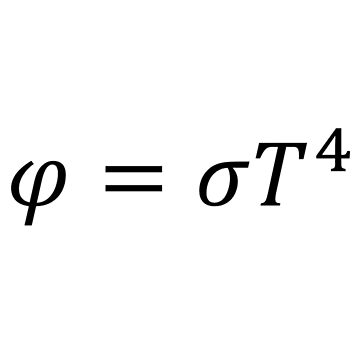The image displays a mathematical equation in black text on a white background. The equation begins with a symbol resembling a cursive or curly "P," which might be the Greek letter phi (φ). Following a space, there is an exceptionally long equal sign, and the rest of the equation continues with a lowercase Greek letter theta (θ), characterized by a circle with a straight line extending to the left from the top of the circle. This is followed by an uppercase italicized "T" raised to the fourth power (T⁴). The spacing between the numbers, letters, and symbols is fairly generous, making the equation clearly legible despite its small font size.